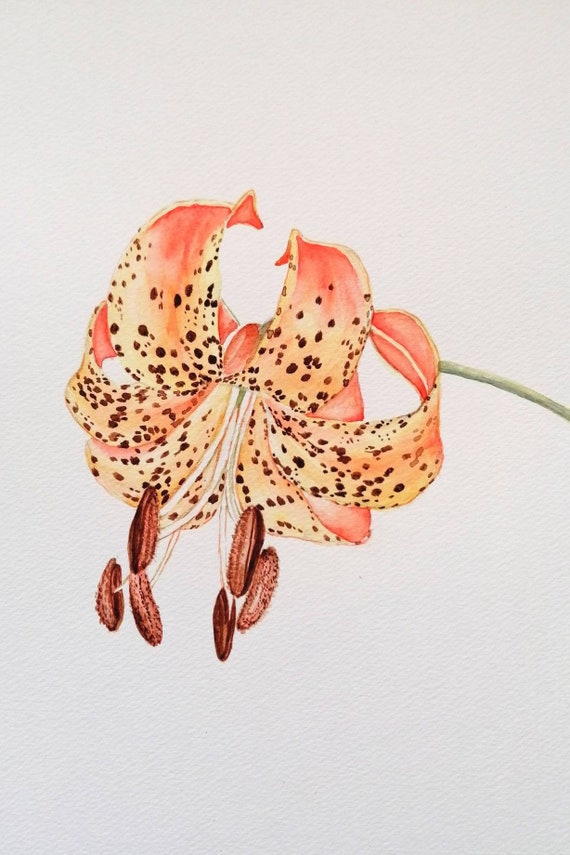This is a highly detailed painting of a tropical flower, meticulously depicted on a plain white canvas. The canvas itself reveals woven ridges, enhancing the artwork's texture. Dominating the center of the image, the flower showcases a single light celery green stem which extends from the right side towards the flower, which has brightly colored petals in shades of orange, coral, and yellow, transitioning to a deep rosy orange. The petals, adorned with sporadic brown spots, curl backward, enhancing their vivid tropical appeal. The flower, resembling a tiger lily, features prominent pistils and stamens that hang down, with three on each side. These stamens have white stems culminating in brown ends. The flower appears slightly downturned, adding a dynamic yet delicate touch to this simplistic and beautiful botanical composition.